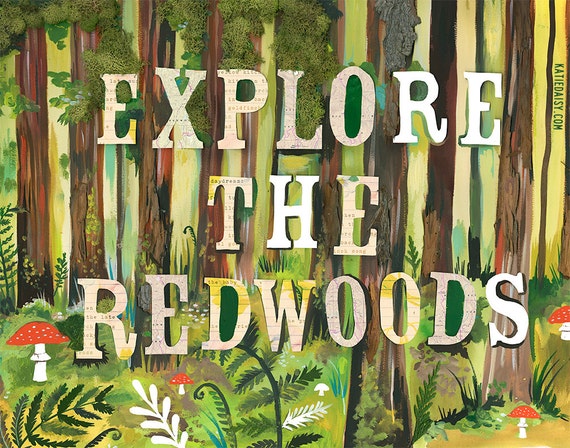The image is a rectangular watercolor artwork, slightly wider than it is tall, featuring a serene and enchanting Redwood Forest scene. Dominating the center in large, capitalized, patterned letters are the words, "EXPLORE THE REDWOODS," creating an inviting call to adventure. Below the text, the forest floor is adorned with lush grass and dotted with four red-capped mushrooms with white stems, adding a whimsical touch. Towering tree trunks form the background, their bark illuminated by hues of yellow, green, dark off-white, and hints of blue, which lend a dreamy, storybook quality to the scene. The tree canopy extends from the top, with leaves gracefully hanging down, completing the picturesque forest ambiance. A subtle element is the vertically rotated text on the right side, reading "katydaisy.com," tying the painting to an artistic context. The overall composition, with its bright, sunny tones and playful, natural elements, evokes the charm of a children's book illustration.